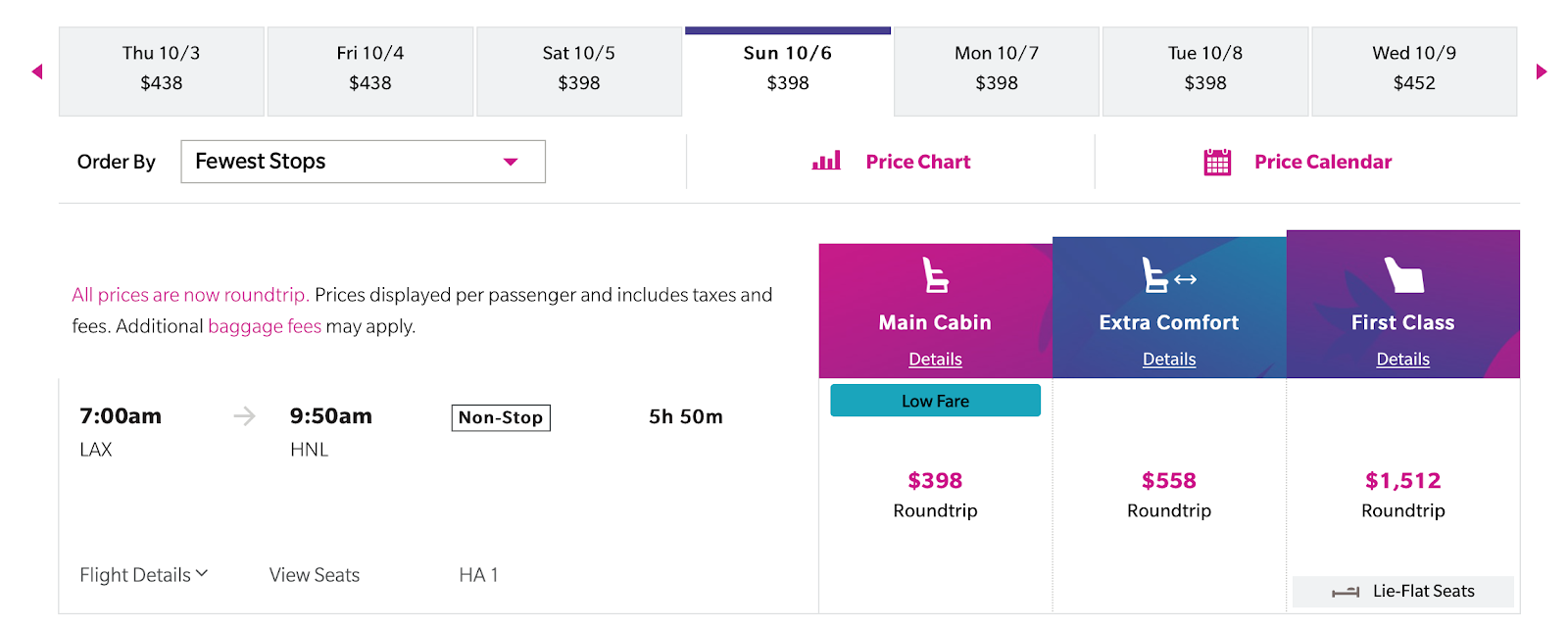This landscape-oriented photo showcases a screenshot from a plane ticket reservation platform, displayed against a primarily white background. The top section features a navigation bar with grey, rectangular date boxes that are slightly longer than they are tall. These boxes display various dates and corresponding prices, flanked by a pink left-pointing arrow on the left side and a right-pointing arrow on the right side, presumably for scrolling through different dates. 

Displayed dates span from Thursday, October 3rd to Wednesday, October 9th, with prices under each date varying — $438, $398, and $452, among others. Below this, on a white background, there's a drop-down menu labeled "Order by" with a pink down arrow, currently set to "few stops." Adjacent to it are two pink icons: a graph labeled "price chart" and a calculator labeled "price calendar." Beneath these options is a pink line of text that states, "All prices are now round trip."

The main content area features three distinct fare options, each on a different color background and progressively taller than the previous one. The options include:

1. **Main Cabin**
2. **Extra Comfort**
3. **First Class** 

Each option lists prices in pink, with First Class being the most expensive at $1,512.